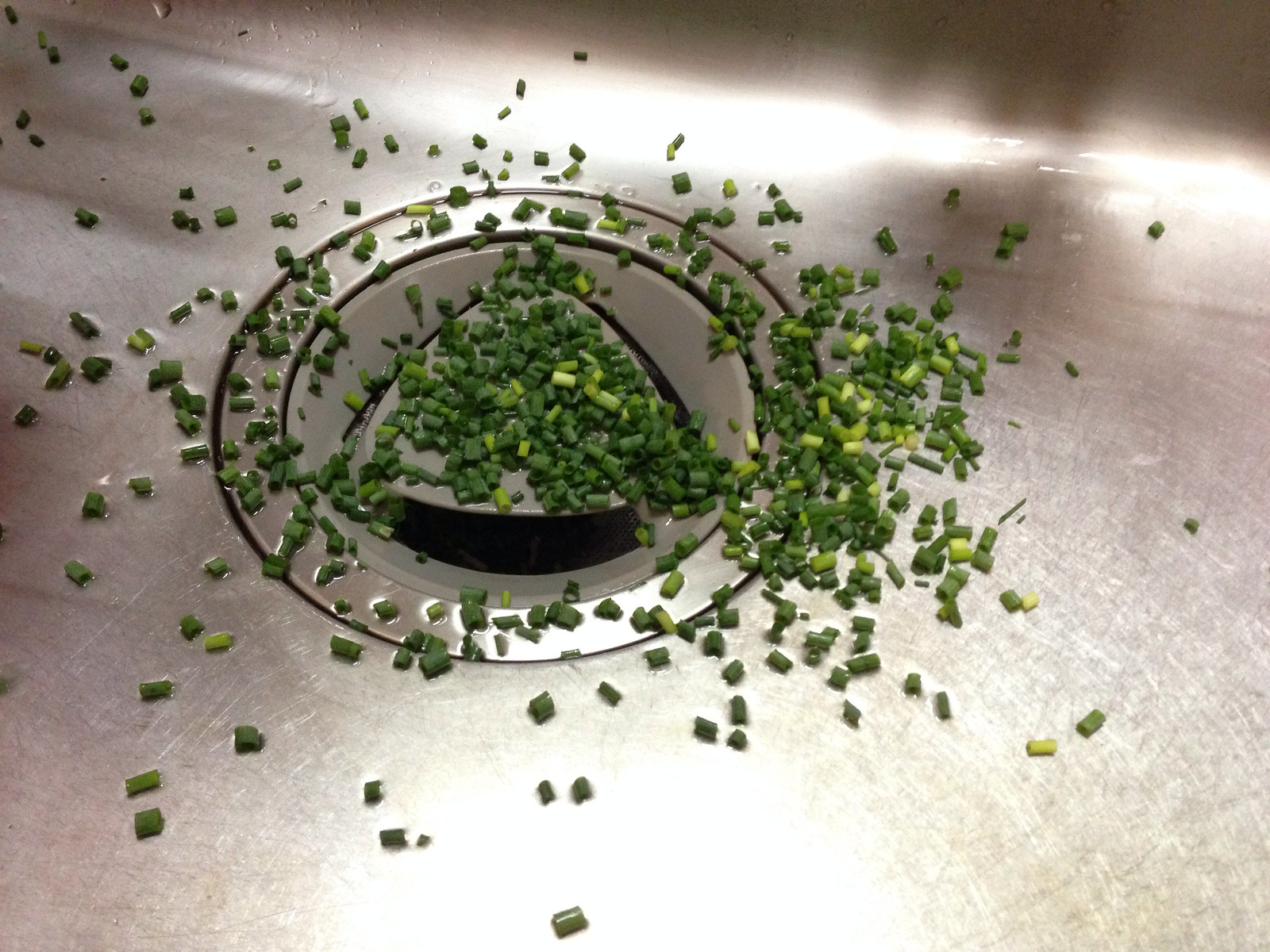This photograph depicts a shiny stainless steel sink, brightly illuminated by an overhead light that creates specular highlights on both the curved walls and the center of the sink. Scattered across the sink, with a notable concentration around the drain, are what appears to be finely diced green onions or chives, numbering in the hundreds. These green pieces cover much of the drain area, forming the largest cluster directly over the drain cover, which is described as a gray plastic piece likely functioning as a drain protector. The sink surface appears slightly wet, enhancing the vibrant green of the chives and the reflective quality of the stainless steel.